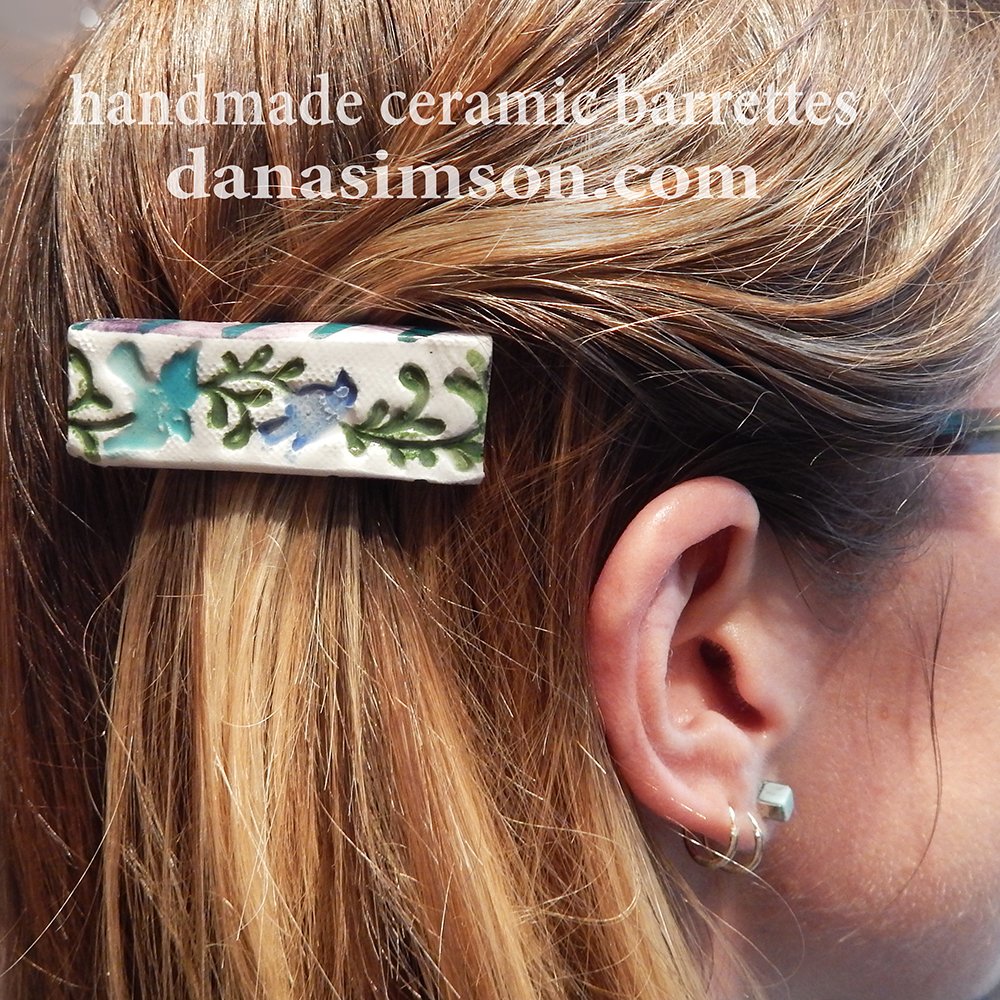The image is a professional promotional photo for handmade ceramic barrettes, featured on the website danasimpson.com. It showcases a detailed, rectangular white ceramic barrette adorned with a delicate floral and bird design in shades of green, light blue, dark blue, and turquoise. The barrette is clipped onto the side of a girl's head, holding her blonde or brunette hair neatly in place. The girl, whose right ear is visible, wears three earrings and glasses, of which only the handle resting on the ear is noticeable. The elegant barrette, combined with her minimalist accessories, creates a stylish and fashionable look.